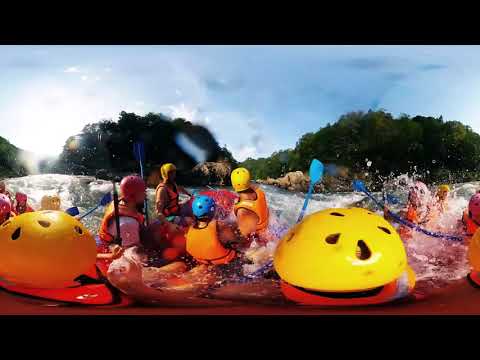The image captures a dynamic, outdoor rafting scene in a vibrant, fisheye-lens perspective, enhanced by a specialized filter. The photograph, bordered by a horizontal black bar at both the top and bottom, showcases several rubber rafts navigating a fast-flowing river surrounded by grassy and tree-lined peninsulas. Each raft, holding approximately four people, is bursting with energy as water splashes vigorously around them. The participants, outfitted in orange or red life jackets, wear helmets in yellow, blue, and red hues, and brandish blue paddles, one of which is raised in mid-air. On either side of the image, large yellow mushroom-like shapes add a curious visual element, while the sun gleams from the left, casting a pronounced glare on the water. The photo, with its vivid realism and detailed freeze-frame effect, captures the rafters leaning back in unison against the forceful waves, immersed in the thrill of their adventure.